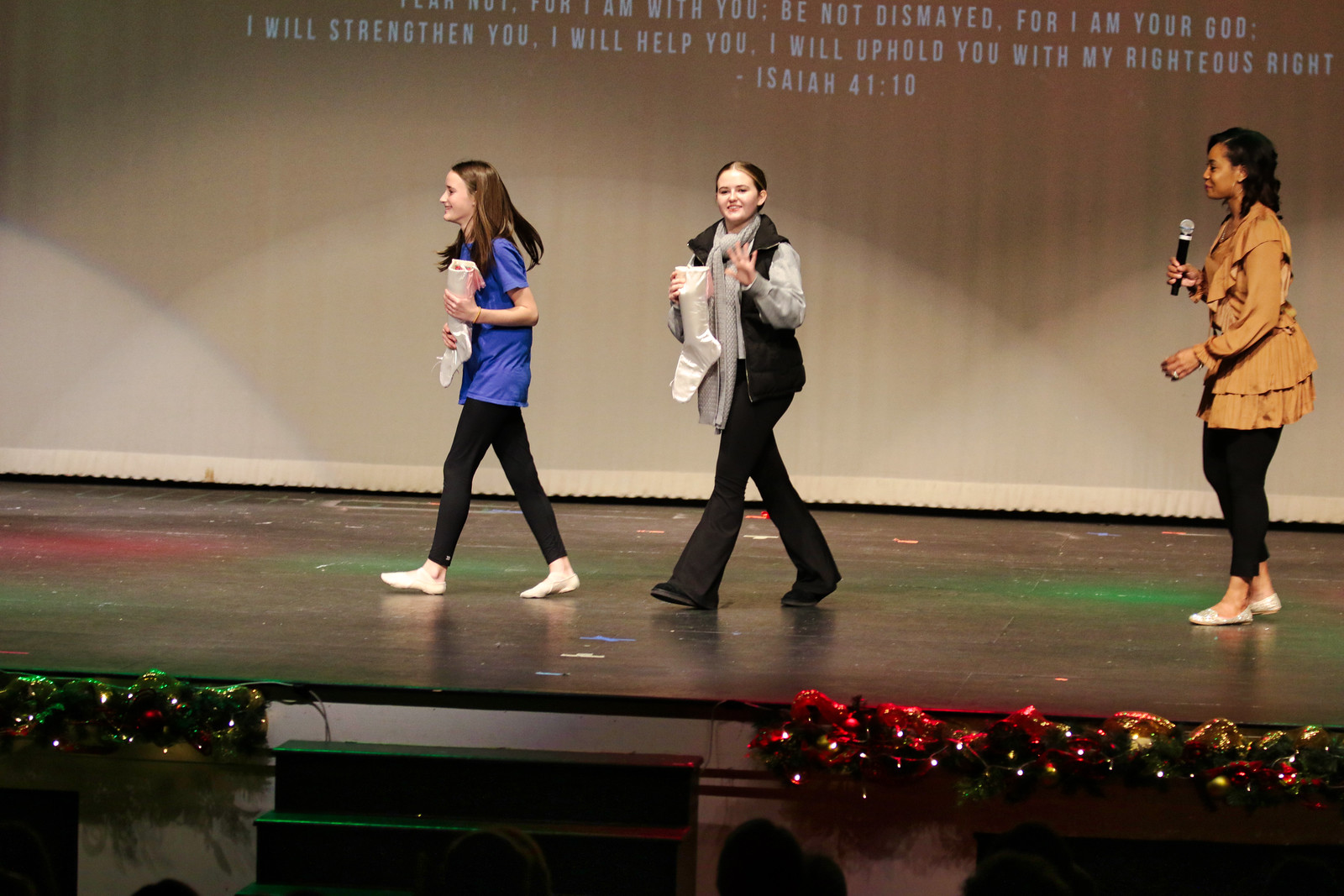The photograph captures a festive scene on a school auditorium stage with a black surface, decorated with evergreen branches and Christmas lights. At the left and center, two young Caucasian girls, likely teenagers, are walking across the stage. The girl on the left is wearing a purple-blue shirt, black tights, and white socks, carrying a white Christmas stocking. She has shoulder-length brunette hair and is smiling at the crowd. The girl next to her, waving at the audience, wears a black vest over a gray shirt, a gray scarf, black pants, and black shoes. She holds another white Christmas stocking in her hand, and her brunette hair is pulled back.

To the right, an older African American woman, possibly a teacher or event organizer, stands with a microphone in her right hand. She dons a yellow-orange shirt, black tights, and white shoes, with long black hair looking towards the girls. Behind them, a projected screen displays a cropped Bible verse from Isaiah 41:10: "Fear not, for I am with you; be not dismayed, for I am your God. I will strengthen you; I will help you; I will uphold you with my righteous right hand..." The heads of the onlooking crowd are visible at the bottom of the image.